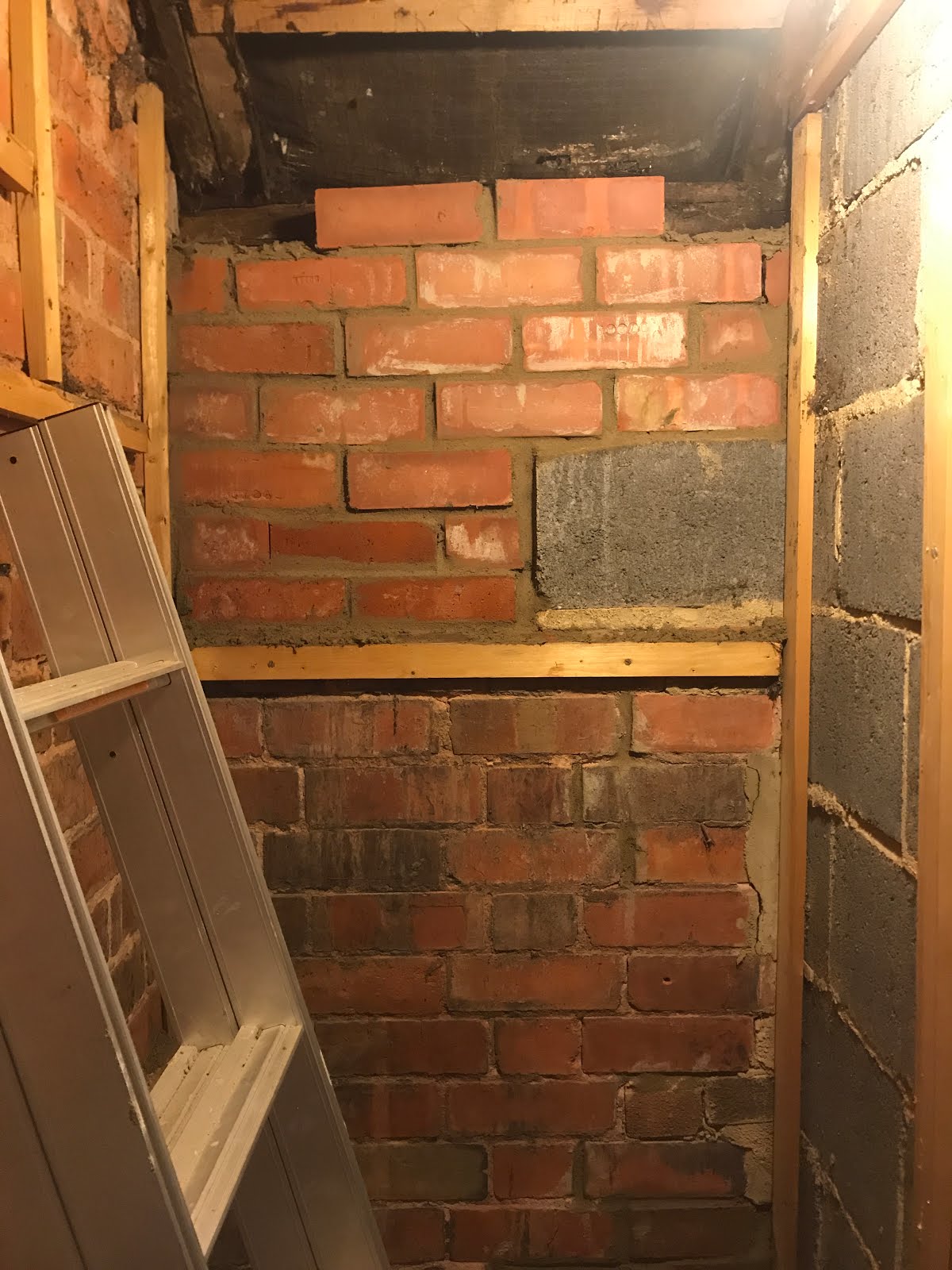The image depicts a very small, closet-sized, space, most likely a basement or an attic, with distinct old construction elements. The left and back walls are made of traditional red bricks featuring dark cement in the back and a lighter cement on the left. The right wall is constructed from cinder blocks with bulging lighter-colored cement. A single cinder block is noticeable near the top of the back wall. A stainless-steel ladder with visible rungs leans against the left wall. Thin wooden strips frame the left and back walls, possibly for future paneling or drywall installation. The ceiling appears to be covered with a black tarp-like material, suggesting ongoing construction or maintenance. The overall setting has a rustic and aged feel, highlighted by the mixed materials and unfinished wooden framework.